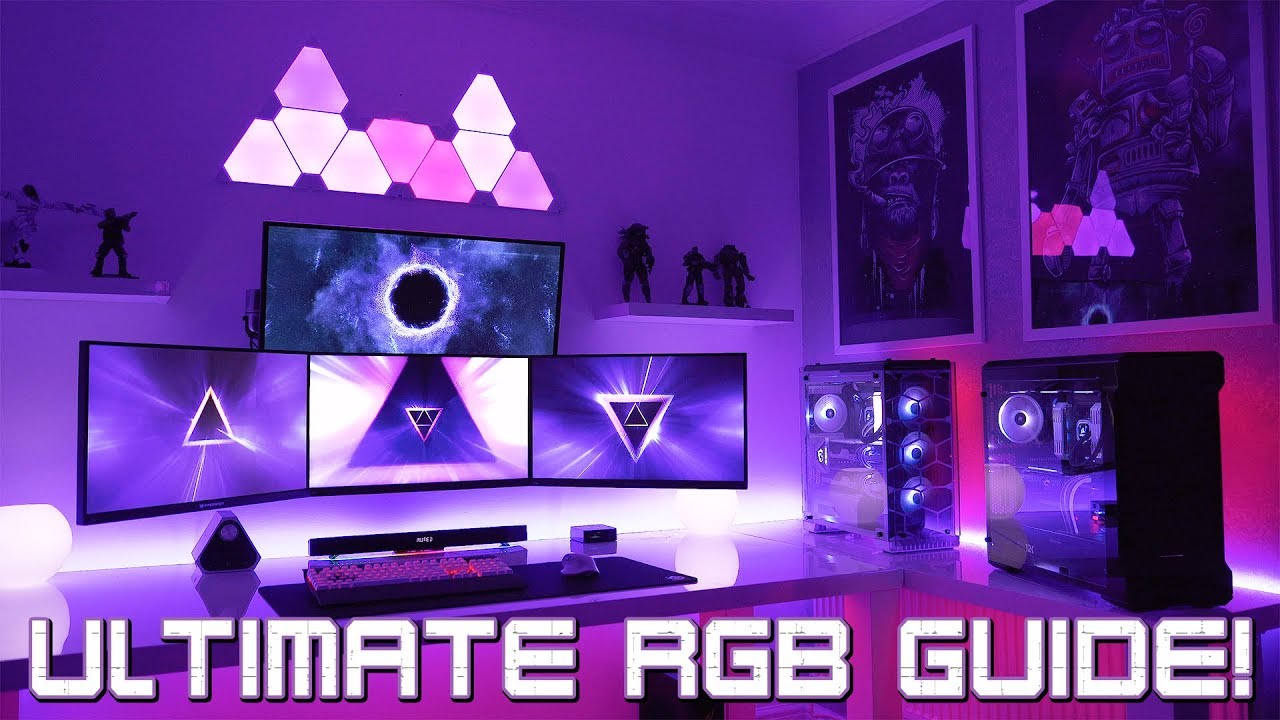The image showcases an impressive and high-tech gaming setup, designed to highlight the ultimate RGB guide. Bathed in a violet and pink glow, the darkened room features a glass-top L-shaped desk adorned with various peripherals, including a wireless mouse, wireless keyboard, black mouse pad, speakers, and a soundbar. Mounted on the wall, four gaming monitors display intricate designs: three show a triangle with rays radiating outward, while the top one has a circular ring with a dark center. The desk is flanked by two RGB-lit desktop towers on the right, positioned under a section of wall adorned with large frames and vibrant NFT-style art pieces, depicting a robot and a monkey smoking a cigarette. Above the monitors, shelves hold figurines, including soldiers, adding a touch of personality to the setup. The entire scene is accentuated by fancy white lighting on the desk and an LED strip behind it, all contributing to a visually stunning and immersive gaming environment. The text at the bottom of the image, displayed in blue, reads "Ultimate RGB Guide."